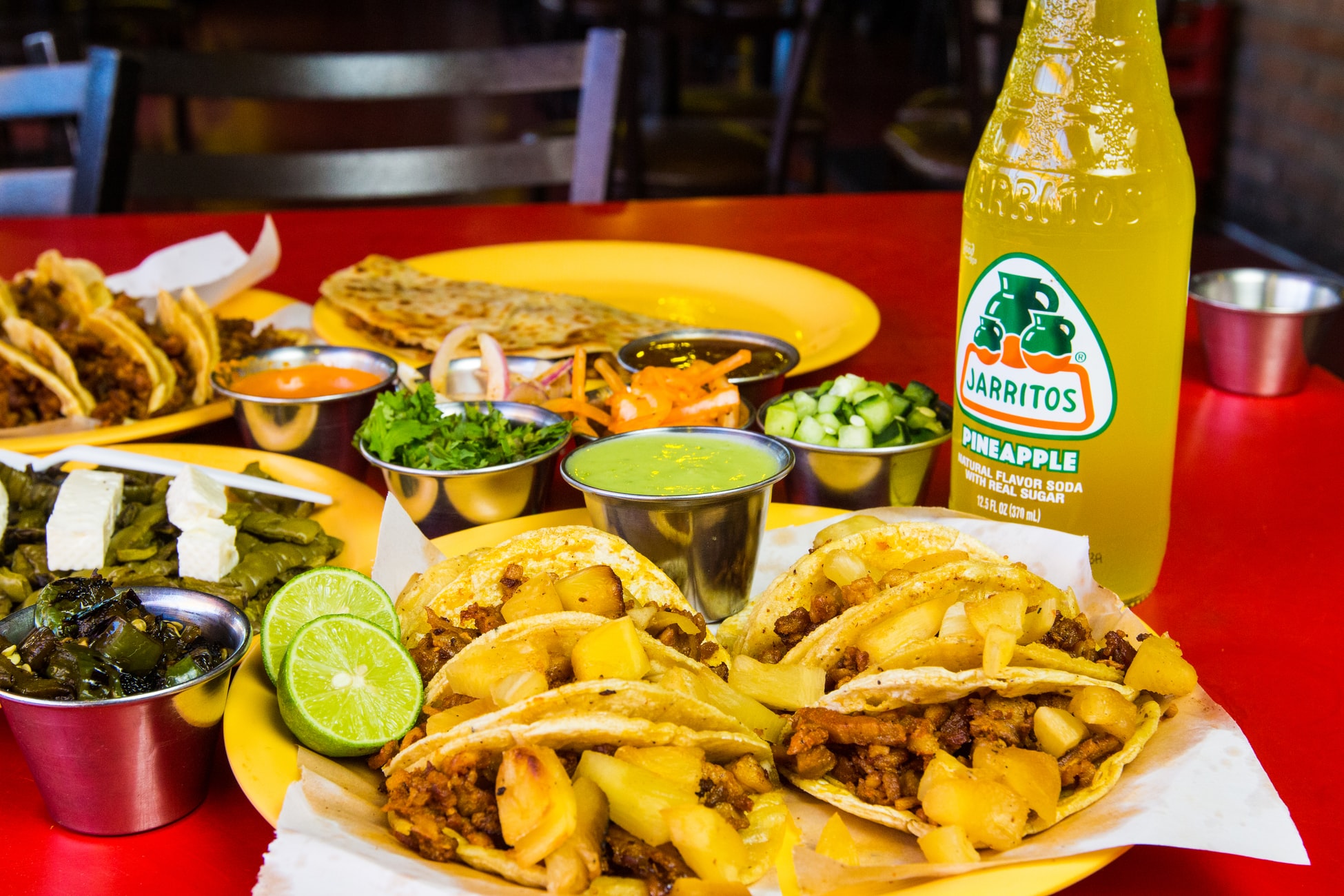This professional product photograph captures a vibrant and inviting scene from a Mexican restaurant, highlighting an array of delectable dishes arranged on a red table. The main attraction is a variety of tacos, likely Tacos El Pastor, served on four yellow plates in the foreground. The tacos, garnished with pieces of succulent pork and accompanied by green Salsa Verde, are bordered by two fresh lime halves. Surrounding them are several silver tins containing diverse toppings and dips, including guacamole, cucumber slices, and other vegetables.

On the left side of the table, there's an interesting mix that appears to be collard greens with tofu, perhaps topped with cheese, along with green beans. These elements add a touch of freshness to the setting. Behind the tacos, there is a neatly folded quesadilla, accompanied by more tacos. Adding to the festive atmosphere, a glass bottle of Jarritos pineapple soda stands prominently to the right, near an empty silver tin.

The table ensemble rests upon a dark red surface, contrasting beautifully with the dark brown wooden chairs in the background. The overall ambiance is enhanced by the view of additional chairs and a stone wall to the right, suggesting a cozy and well-appointed dining area.